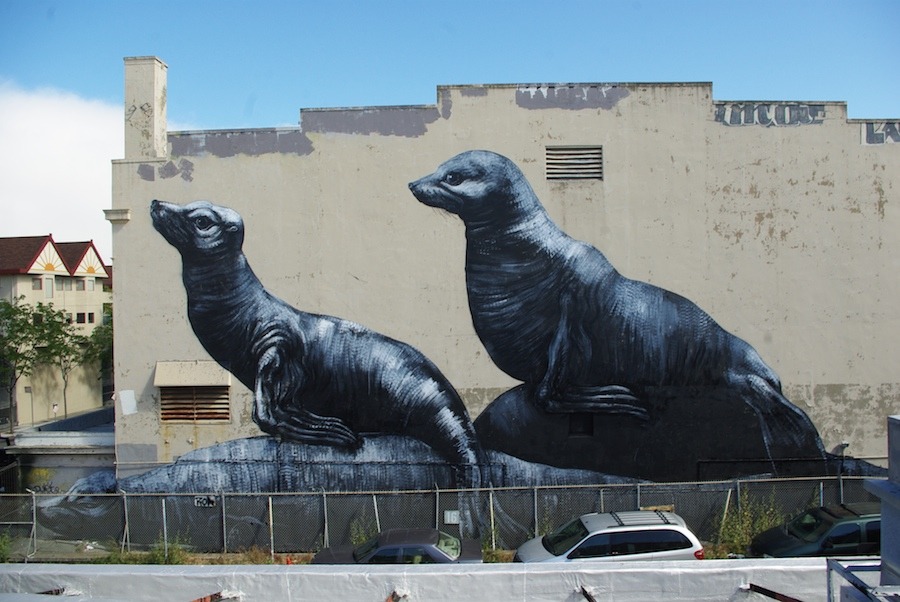This is an outdoor photograph of a striking mural painted on the side of a large, somewhat oddly-shaped but overall rectangular tan building. The mural vividly depicts three dark gray sea lions with white accents. One sea lion is lying down on a rock, while a smaller one is perched on its back, and a third sea lion is positioned next to and behind them. All three sea lions are gazing towards the left side of the image. The building also features two vents; one located just below the sea lion with the oddly shaped head, and the other behind the second sea lion. There is a visible chimney to the left side of the building. Directly in front of the mural is a chain-link fence with three cars parked along it. To the left of the mural, there is a townhouse building. In the background, other homes and trees are visible along with rooftops featuring sun designs. The photograph captures a bright, sunny day with a blue sky dotted with a few low-lying white clouds, and seems to have been taken from the roof of an adjoining building, as a wall and some equipment are visible in the foreground.